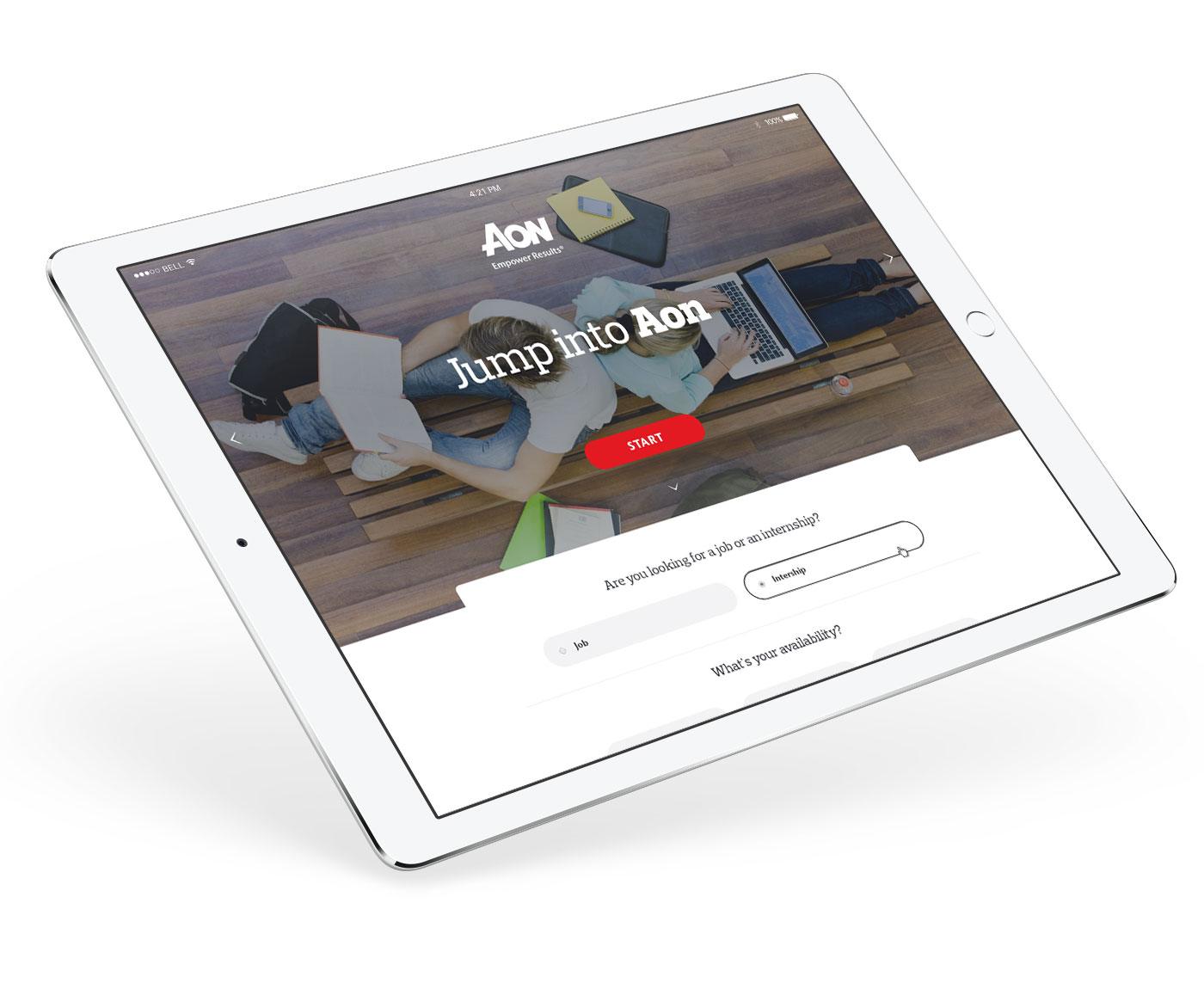The image appears to be a screenshot of a website, presented on a white background with the appearance of a slightly diagonal, square-shaped tablet. The device casts a slight shadow underneath, giving the impression that it is tilted and resting on its lower left corner. The tablet features a white edge and displays several icons at the top, including an unreadable time in the center, a battery icon on the right, and additional icons on the left.

Prominently, the screen shows a greyscale image of two individuals sitting on a bench. The person on the right is using a laptop, while the person on the left is reading a book. Below this image, the text reads "Aeon. Jump into Aeon," along with a striking red "Start" button. Further down, there's a question hinting at a job or internship opportunity: "Are you looking to...?" with more content that seems related to internships.

The interface also contains two rounded rectangles, with a cursor hovering over the one on the right. Although the text inside these rectangles is too small to decipher, the underneath text asks about the viewer's availability. Scattered books and bags around the bench suggest that the ad targets students, likely those seeking internships or job opportunities.